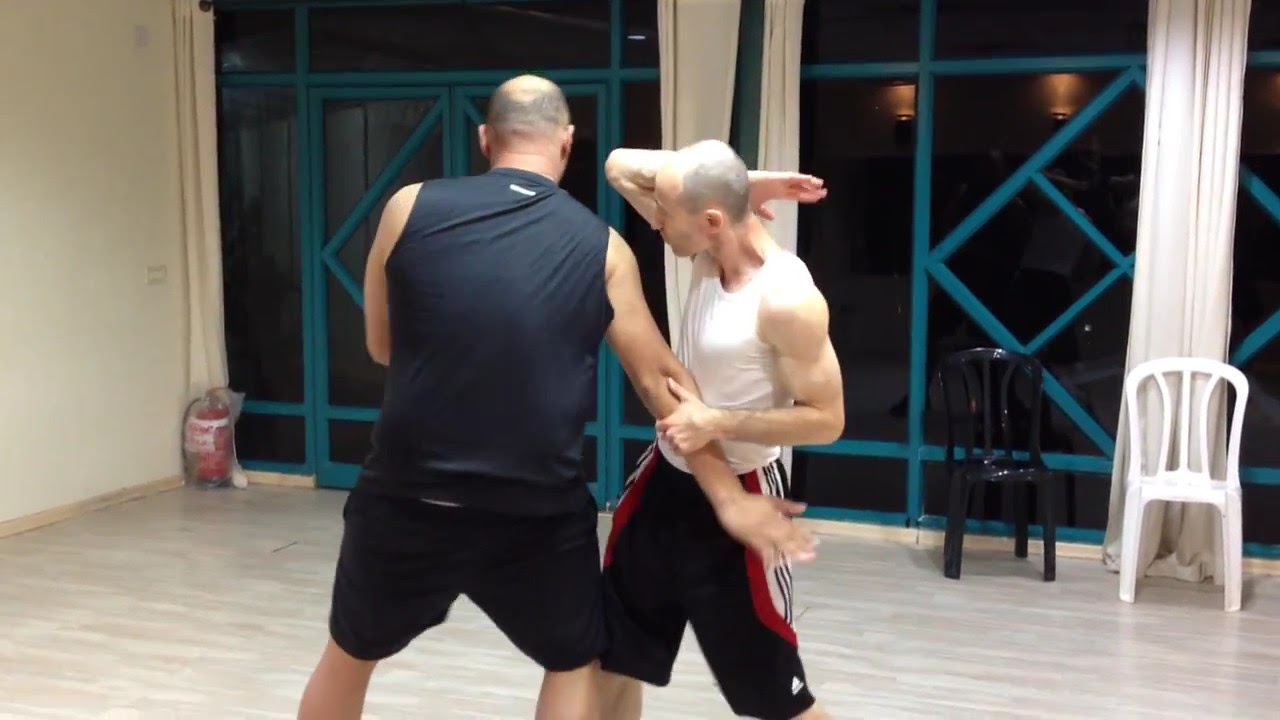The image shows an indoor gym or dance space with a light-colored, almost white-gray wooden floor. Two men are prominently featured, seemingly engaged in a martial arts lesson. On the left, a slightly older man with balding gray hair is seen from behind. He wears a black sleeveless top and black shorts, with his right arm extended downward, being grasped by the other man. This other man, who is smaller, muscular, and wearing a sleeveless white shirt with black, red, and white shorts, appears to be demonstrating a move. His body faces towards us, with his left arm gripping the older man's forearm and his right arm bent at the elbow, positioned behind his head. The background features a large window with blue beams for support, a black wall with white curtains, and two plastic chairs—one black and one white—positioned to the right. A fire extinguisher rests in the left corner, completing the scene with an emphasis on space and safety.